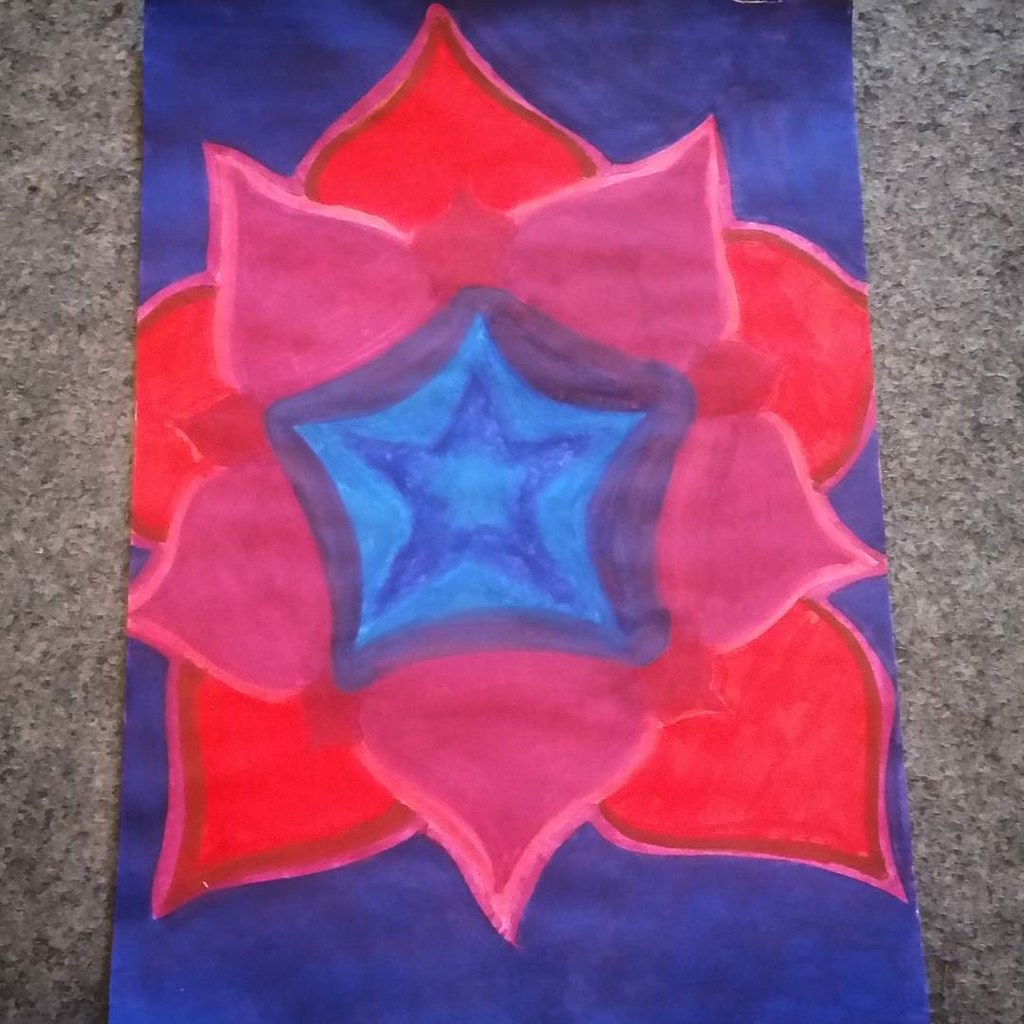This nearly square image captures a handmade card, positioned vertically on a granite tabletop. The card dominates the frame, with only narrow strips of the granite surface visible on the left and right edges. The card itself features an intricate design at its center: a dark blue star set within a pentagonal shape, surrounded by a lighter blue area. Extending from this central star are five pink, leaf-like petals with lighter pink edges. Behind these are five staggered, rounded petals, colored in red with darker red outlines. The background of this striking flower design is a rich dark blue, complementing the central star and enhancing the overall visual appeal of the card.